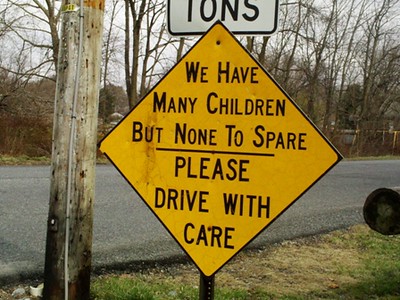This image captures an angled view of a triangular yellow sign with a thin black border and black lettering that reads, "We have many children, but none to spare. Please drive with care." Positioned above this sign is a rectangular white sign with black text indicating the weight limit for vehicles ("tons sign"). To the left of the signs stands a wooden light pole with visible wires running vertically along its length. In the background, there is a mix of grassy areas and an asphalt road that extends diagonally from the bottom left to the center right of the image. The scene is framed by leafless trees lining the opposite side of the road, emphasizing a stark, wintry landscape.